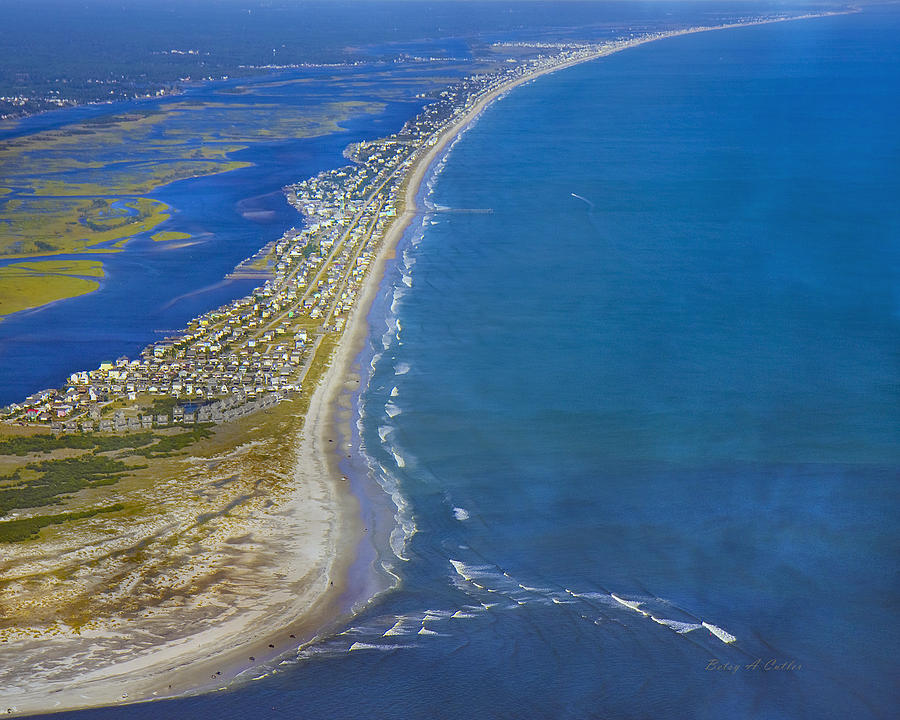This aerial photograph captures a strikingly large body of bright blue ocean, interspersed with several landmasses. The main feature is an exceptionally long strip of sandy beach that starts out rounded and bulbous at the bottom and tapers into a fine line as it extends far into the distance. The land strip is populated with a variety of buildings—some possibly commercial or residential, sporting colors like white, gray, and blue, giving it the appearance of a developing subdivision or a small metropolitan area. The landscape includes patches of grass or greenery, enhancing the visual contrast against the sandy shore. Smaller green islands are scattered within the ocean expanse, adding texture to the predominantly blue scene. In the corner, a larger, darker mainland area appears blurry. The image, likely captured from a high altitude via drone or airplane, offers a comprehensive, overhead view where approximately 70% of the frame is dominated by water, accentuating the vastness and beauty of the oceanic environment.